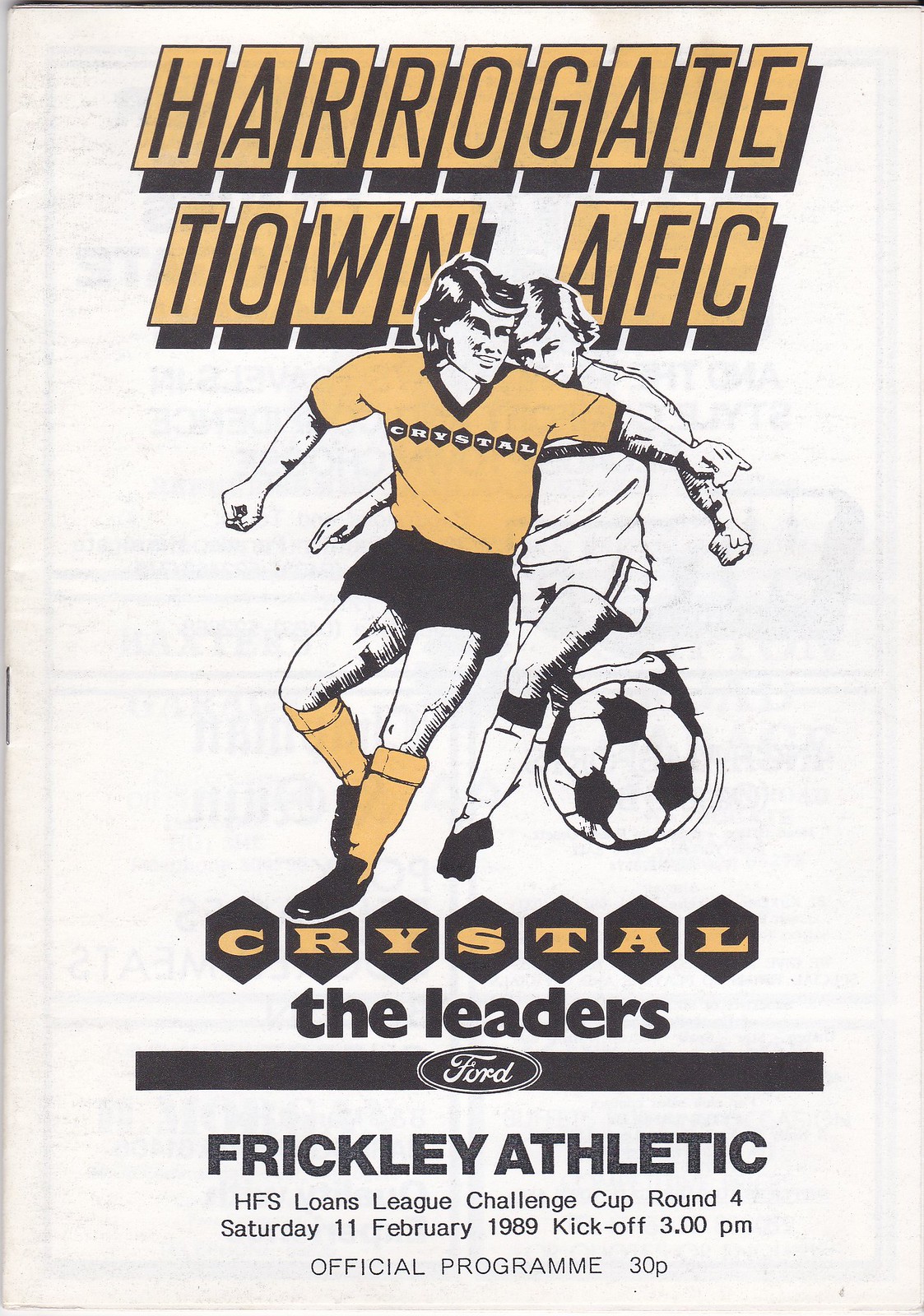The front cover of the soccer program showcases a clean white background. At the top, bold black letters spell out "Harrogate" set against individual orange squares outlined in black, complete with a subtle black shadow effect behind each letter. Just beneath, more orange squares spell out "Town A.F.C" in black letters. Below this heading, a black and white illustration features two soccer players, one wearing an orange jersey with black shorts and the other in a white shirt with white shorts, with a soccer ball positioned between the legs of the player in white. Moving further down, the word "Crystal" is prominently displayed in orange letters within black diamond shapes. Below "Crystal," the phrase "the leaders" appears alongside a black horizontal bar that prominently features the Ford symbol at its center. Further down, the program indicates "Frickley Athletic, HFS Loans League Challenge Cup, Round 4, Saturday, 11 February 1989, kickoff 3 p.m." It completes with "Official Program 30p" at the very bottom.